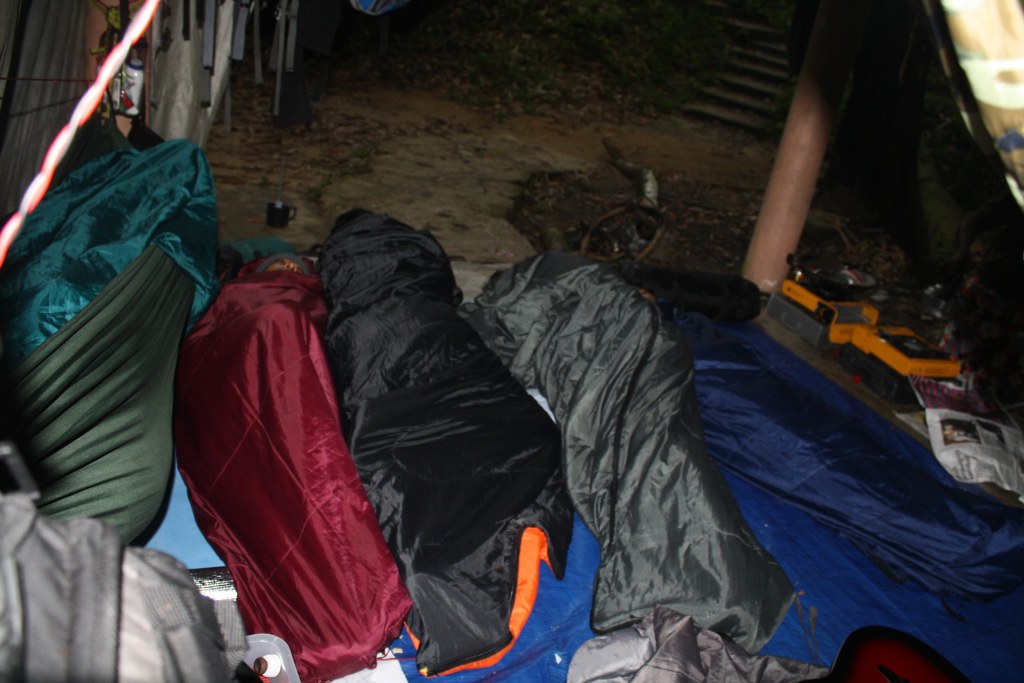The photograph depicts a somber outdoor scene taken from an overhead perspective at night, revealing a group of individuals sleeping on a blue tarp laid over a dirt ground. The dim lighting adds to the melancholy atmosphere, casting shadows over the array of vibrant sleeping bags in various colors: a medium blue, gray, green, black with an orange interior, and burgundy. Notably, the only visible face is of the person in the burgundy sleeping bag, who is wearing a green ski cap. 

Scattered around the makeshift beds, there are assorted personal items and debris, suggesting a transient or homeless community. A closer inspection reveals more details: balled-up sheets and blankets in a variety of hues including green, turquoise, magenta, black, gray, blue, and orange dominate the front of the scene. A gray backpack is also present, possibly holding more belongings. In the background, a set of steps leads downward, indicating the group is sheltered under some structure. To the right of the image, a black coffee cup, a brown guitar's edge, a newspaper, and some bright yellow camping heating elements stand out amidst the dimness, adding to the tableau of a tough, possibly homeless life.